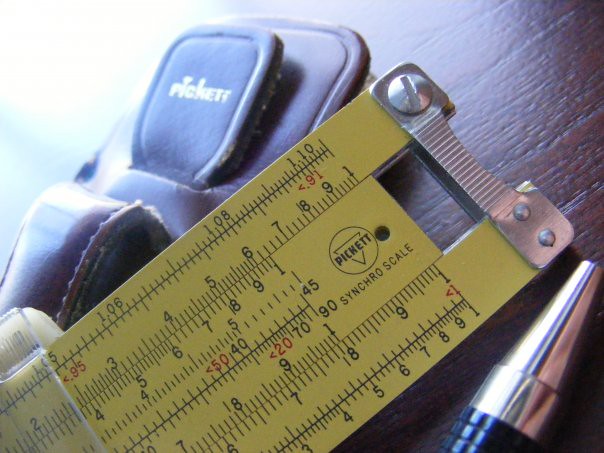The photograph captures an assortment of tools meticulously arranged on a rustic wooden desk. Dominating the left-rear of the image is a leather pouch or tool holder, subtly illuminated by light seeping in from the corner, partially obscuring some of its details. The pouch appears to have text etched in white, possibly reading "Picket" or "Ricket." Centered prominently in the frame is a vivid yellow tape measure, replete with black markings, numbers, and detailed indentation lines that lend an air of precision to the scene. This measuring tool boasts a metallic edge and is secured with a couple of visible screws. To the bottom right, the tip of a pen peeks into the frame, adding a final touch to the composition of tools, suggesting meticulous readiness for work.